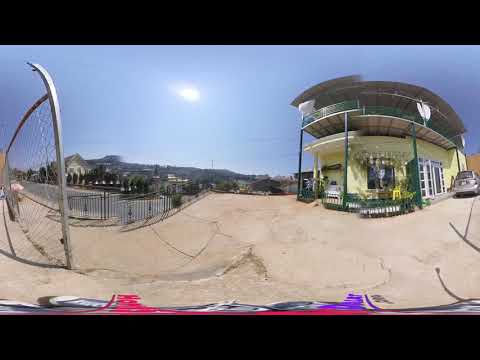In this clear, sunny daytime image, framed against a backdrop of blue skies without any clouds, we see an exterior suburban scene that seems to combine elements of a skate park and a parking lot. Dominating the center is a bright yellow building, possibly a small hotel or house, featuring a green awning or balcony that hints at a Mediterranean architectural style. A silver car is parked next to this building, and there are a few other cars in the distance. The ground appears deserted, though a person can be seen walking behind a fence to the left of the image, near a street. Inscribed graffiti on the ground suggests this might be a part of a skate park. In the distant background, the cityscape and rolling hills add depth to the panoramic and slightly distorted 360-degree photo. The setting looks fenced off, possibly indicating a private area, and the overall scene appears calm and peaceful under the bright sun.